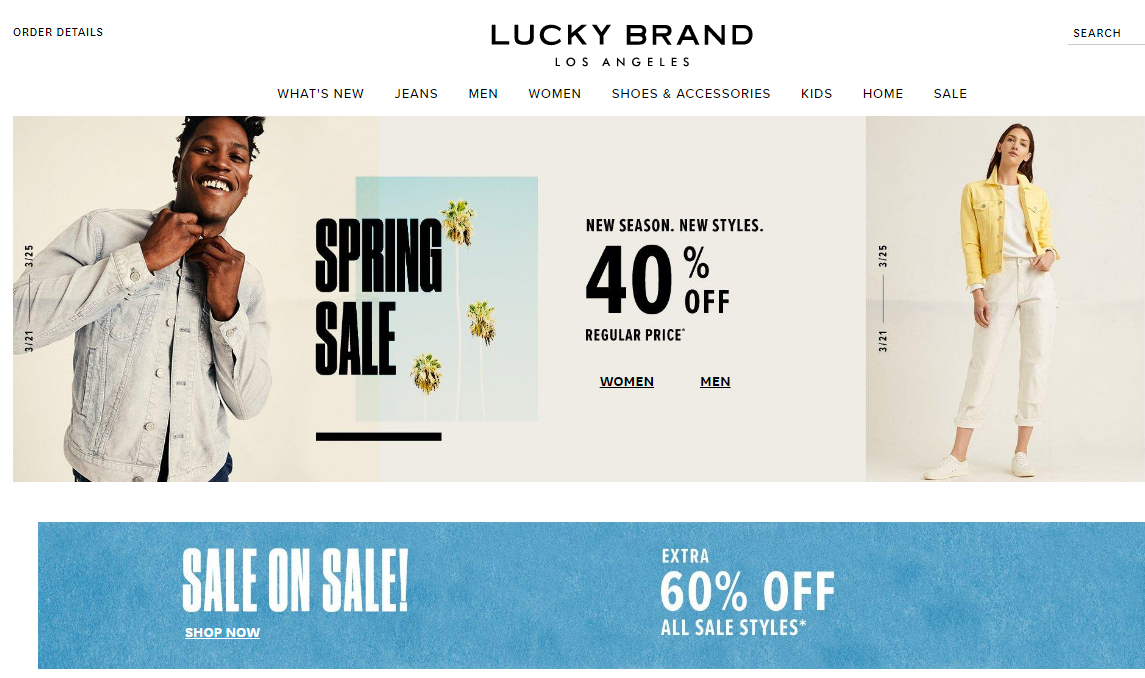A screenshot from the Lucky Brand Los Angeles website announces a "Spring Sale: 40% Off New Season, New Styles." The promotion targets both men's and women's collections with a regular price. On the left side of the image, a Black male model is shown buttoning up a stonewashed denim jacket. On the right, an Asian female model features a confident stance with one hand on her hip, wearing white trousers, white shoes, and a stylish white and yellow blazer. The backdrop is a subtle cream color. At the bottom, a blue banner highlights an additional "Extra 60% Off All Sale Styles," with a "Shop Now" call-to-action button.